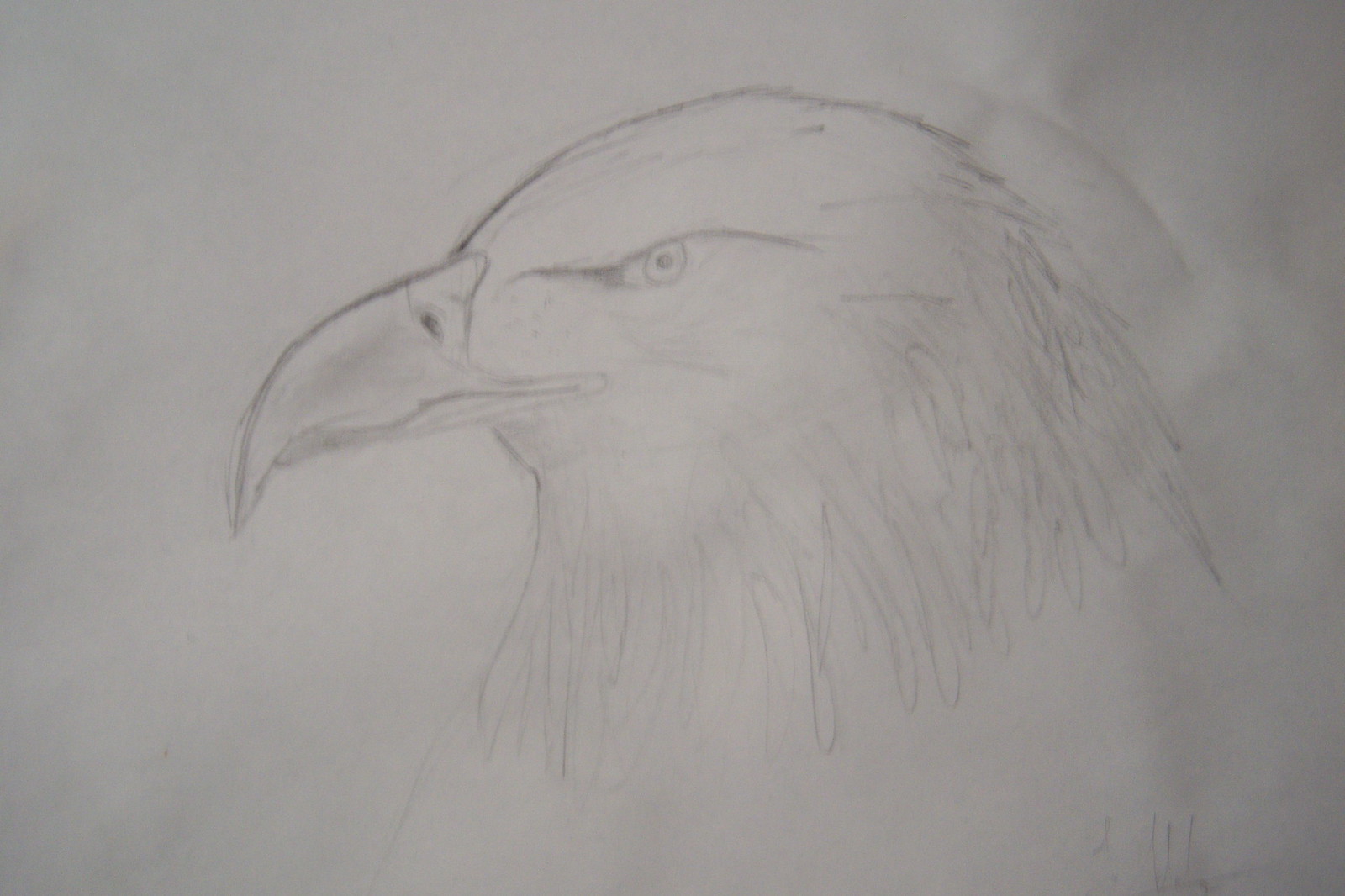This close-up photograph captures a detailed pencil drawing of a bald eagle's head sketched on white drawing paper, which shows crinkling and wrinkling on the right side. The drawing is black and white, rendered entirely with pencil, and exhibits no use of colored materials. The eagle's head is predominantly white, emphasizing its identity as a bald eagle. The piercing eye, expressing a sense of anger, features a dark black line above it. The eye itself is an oval shape with a smaller, shaded circle representing the pupil. The beak is illustrated with a pointy tip, shaded in light gray, with a small black-shaded circle near the face and a darker gray line indicating the mouth. The feathers are intricately drawn, employing wisps and zigzag patterns to showcase texture and detail. The image shows the head in side profile, and although the background paper appears white, slight variations or variegations in shading might give it a subtly darker appearance in certain areas.